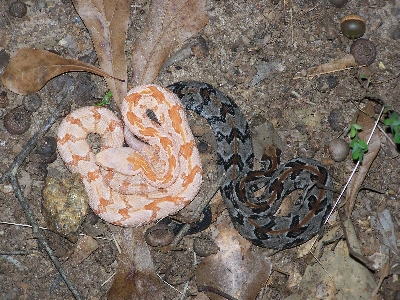This aerial photograph captures a forest floor strewn with dead leaves, acorns, and small rocks against a backdrop of brown ground. Two snakes, both curled yet distinct in appearance, are the focal points. On the left coils a white snake with striking orange chevron markings, reminiscent of sherbet, possibly an albino species. Its head rests prominently on top of its body. To the right lies a gray snake adorned with black markings and a brown stripe running down its length, showcasing a more extended, less coiled posture compared to its neighbor. The two snakes, although in close proximity, do not intertwine. Their surroundings—a natural mix of dirt, dried leaves, sticks, and acorn shells—suggest a wild landscape, capturing a serene, unspoiled moment in nature.